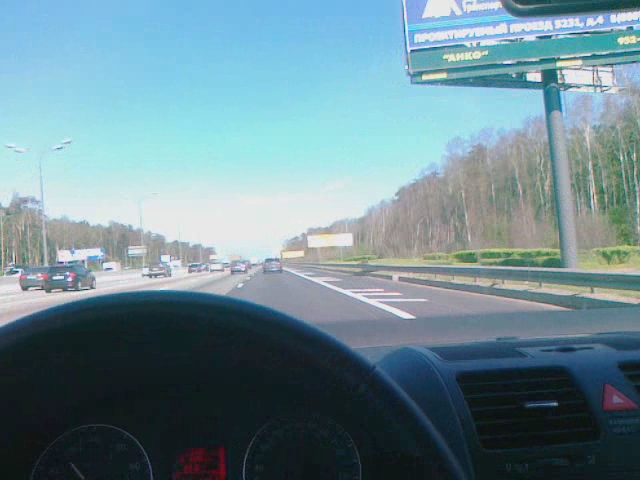This daytime photograph captures the view from the driver’s seat of a car, looking out through the windshield onto a bustling four-lane interstate. The interior of the car features a sleek black steering wheel and dashboard, with only the top portion of the speedometer and AC vents visible. Beyond the dashboard, the busy interstate is separated by a concrete divider, with traffic flowing in the opposite direction on the other side.

To the right of the interstate, a large, elevated billboard is visible, though only the bottom part can be read, and it blurrily displays the letters "A H K O" and the number "952". The scene suggests a slightly chilly time of year, evident from the bare trees lining the roadside, although patches of green shrubbery are also visible on the right shoulder of the highway.